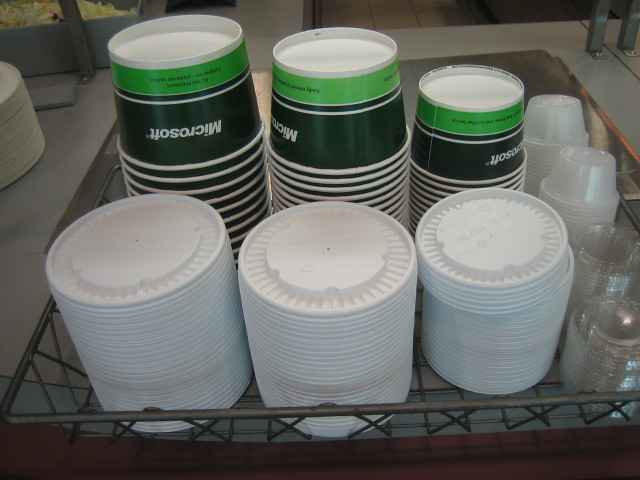The image captures a commercial setting with a large metal rack holding multiple stacks of navy blue paper bowls, all emblazoned with the word "Microsoft" and accented by a strip of green around the bottom. These bowls, stacked upside down, appear in various sizes—large, medium, and small—with corresponding white lids placed in front of each stack. Additionally, there are two rows of smaller, clear plastic sauce containers and their lids positioned in front, intended for condiments like ketchup. The scene conveys an organized layout, suggesting the bowls are possibly intended for carrying soups or other liquids, contributing to a well-prepared carry-out station in a commercial kitchen or similar environment.